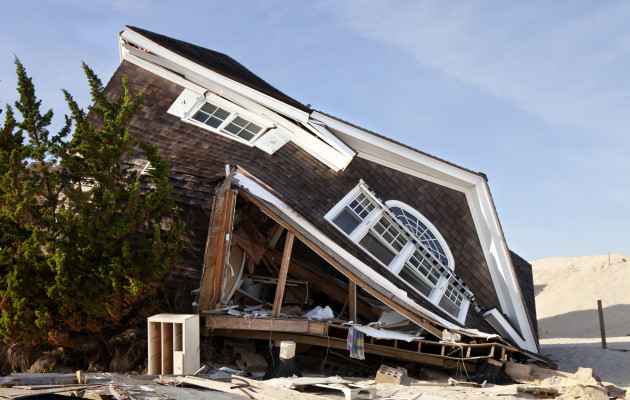The image, a color photograph in landscape orientation, captures a detailed view of a large, dark brown shingle house with white trim and a dark, triangular-shaped roof that has collapsed, likely due to an earthquake or natural calamity such as Superstorm Sandy in New Jersey. The house is extensively damaged, with the left side somewhat intact while the right side has tilted down into the sand below, revealing a demolished wooden porch and a destroyed foundation. The scene is set against a backdrop of a clear, pale blue sky with scant white clouds, and sunlight illuminating the surroundings. The area around the house features a hilly landscape with sand, a tree on the left, and the absence of grass, suggesting an open field. The photograph employs a style of photographic representationalism and realism, effectively conveying the scene's post-disaster desolation.